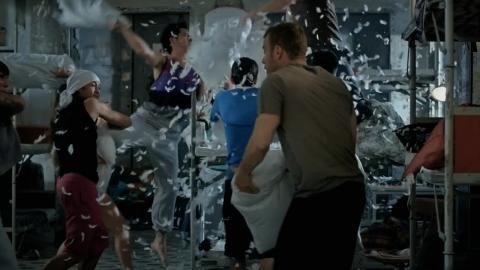The image captures a lively and chaotic pillow fight involving six people in what appears to be a large room that could be a dormitory, possibly military barracks. The scene is filled with flying feathers, likely from burst pillows, adding to the frenzied atmosphere. The central figure, a man wearing an olive green t-shirt and black pants, is prominently positioned and appears to be pulling a pillow out of its case, gearing up for the next strike. To his left, a woman in a blue shirt faces away from the camera, participating in the action. The room features metal bunk beds with white mattresses, pipes, and a chalkboard in the background, suggesting a utilitarian setting. Colors in the image include shades of white, black, purple, gray, red, blue, and brown. Despite the dynamic activity, no one's face is fully visible, obscured either by their positions or the swirling feathers. The sense of motion is palpable, with participants caught mid-action, some jumping, others mid-throw, contributing to the vibrant, playful chaos of the scene.